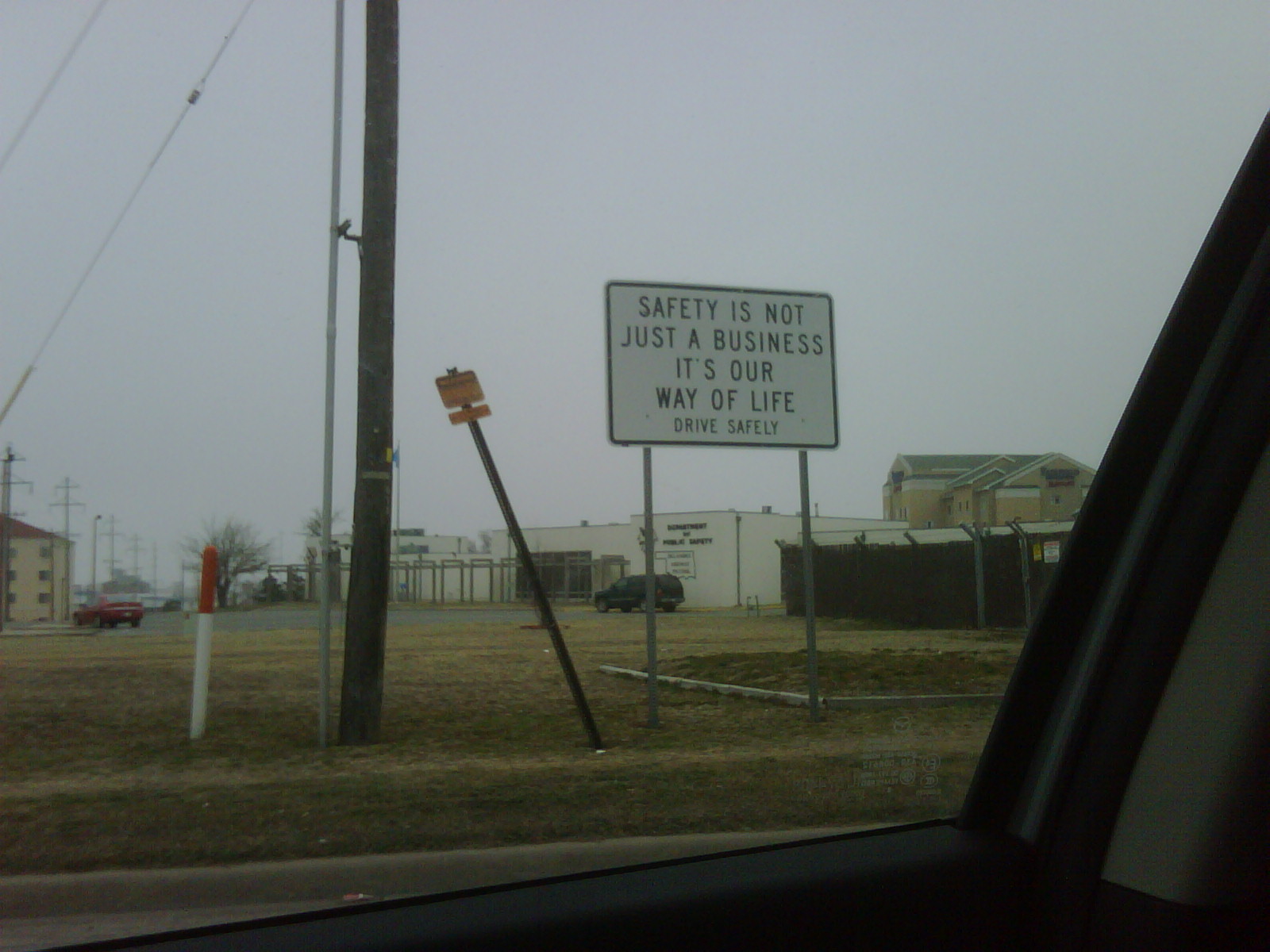The photograph, taken from the passenger side of a vehicle, captures a dreary scene on a rainy day. It prominently features a large, white, rectangular sign attached to two silver posts, bearing the message: "Safety is not just a business, it's our way of life. Drive safely." This sign is the centerpiece of the image. To the left of this sign, a smaller yellow sign is seen leaning on a black stake, likely having been struck by a vehicle. The foreground includes various elements of the car's interior, with visible portions of the door frame in black and green, and some lines or wires in the top left corner. A wooden telephone pole stands adjacent to a metal pole in the background. The scene is set against a backdrop of multiple buildings: a white office-like building centrally located, a possible hotel building situated further behind, and a red apartment building with windows to the left, complete with a red car parked nearby. Additionally, a short white and orange pole is planted in the ground on the left side, and several other vehicles are parked in a fenced area around the buildings. The sky is gray and overcast, adding to the overall gloomy atmosphere of the photo.